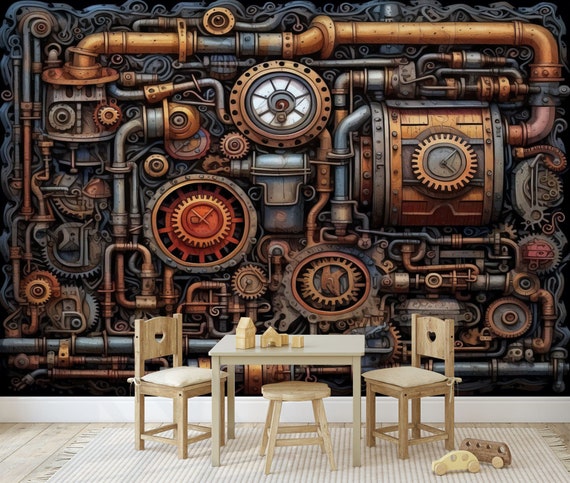The image showcases an artistic rendering of a whimsical children’s room with a steampunk twist. The focal point is an intricate, steampunk-inspired wall composed of interconnected gears, pipes, and valves in hues of gold, copper, silver, and red, complete with embedded clocks and machinery. The remainder of the room contrasts this industrial backdrop, featuring a quaint setup of children’s furniture. A small, light brown wooden table is centrally placed, flanked by two matching chairs, each adorably adorned with heart cut-outs on the backrests, and a wooden stool tucked beneath the table. The tabletop is dotted with wooden toys, including miniature houses and building blocks, while the floor below, covered by a light-colored rug with white and gray stripes and tassels, holds an assortment of wooden cars and buses. Overall, the scene blends the mechanical complexity of the steampunk wall with the cozy, playful simplicity of a child’s playroom.